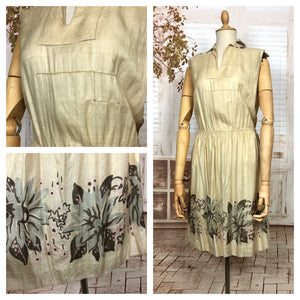This image showcases a light brownish khaki or beige dress displayed on a headless mannequin, likely in a store with tile flooring. The dress, reminiscent of an apron design, is short-sleeved with a modest opening at the top. Detailed black and gray floral embroidery adorns the lower third of the dress, which is highlighted in a close-up image. The image appears to be a composite, resembling a kaleidoscope view, with three distinct sections: a full view of the dress, a focus on the top half, and a close-up of the embroidered floral design at the bottom. This detailed presentation suggests it might be used as an advertisement to showcase the dress.